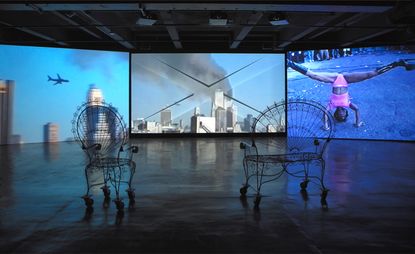This image is a dark, indoor photograph captured in landscape format, likely an art installation set within a studio or warehouse-like space. In the foreground, there are two garden chairs constructed of steel rods, designed in such a way that one can see through them. These chairs are placed to face three extremely large monitors at the far end of the room and seem to sit atop a glossy black floor. The room has a dark ceiling with numerous horizontal and vertical bars, from which three lights hang unlit in the top middle area. The scene feels very dimly lit, adding to the overall somber atmosphere. 

The leftmost monitor shows an airplane approaching the World Trade Center, with clear impending impact. The central monitor depicts the aftermath, with thick smoke billowing from the Twin Towers, capturing the catastrophic events post-crash. The rightmost monitor diverges drastically in theme, displaying a woman doing a headstand on a street. She is dressed in a pink top and pink underwear worn on her head, with her legs extended in a split and adorned with black knee-high high-heeled boots. The overall composition of the photograph suggests a juxtaposition of catastrophic historical events with an eccentric, almost surreal, human activity, against a backdrop that enhances the poignancy and oddity of the scenes.